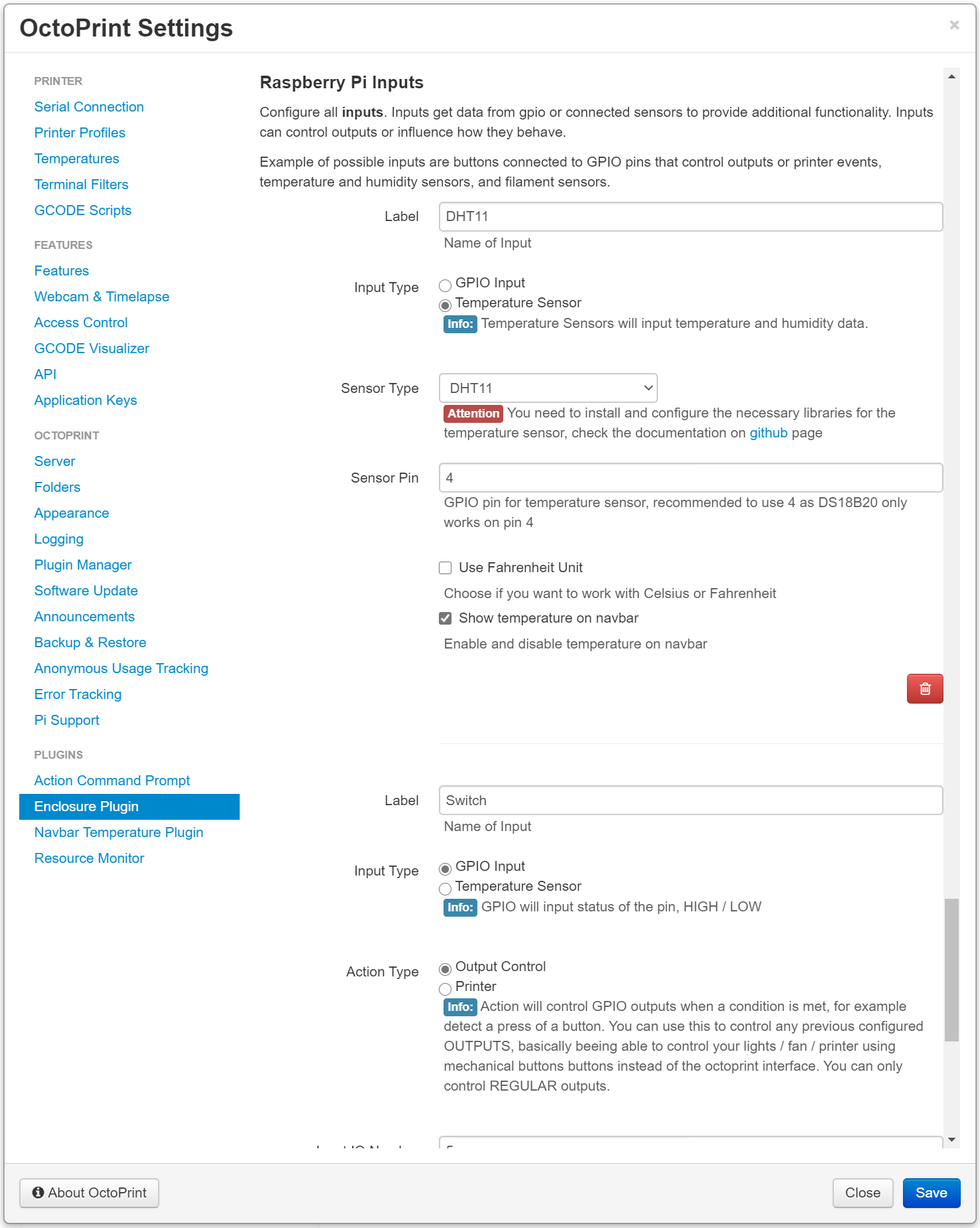This screenshot captures a comprehensive view of the OctoPrint Settings window. Dominating the upper part of the window is the title, "OctoPrint Settings." The left side features a vertical menu bar divided into multiple sections: Printer, Features, OctoPrint, and Plugins. The currently highlighted menu item is the Enclosure Plugin, which is located under the Plugins section. The right side of the window displays detailed information specific to the Enclosure Plugin. At the top of this section, the header reads "Raspberry Pi Inputs," followed by thorough instructions and guidelines on how to configure these inputs. The content includes extensive text and appears to involve elements specific to coding or computer networking, indicating advanced customization or control settings for the Enclosure Plugin.